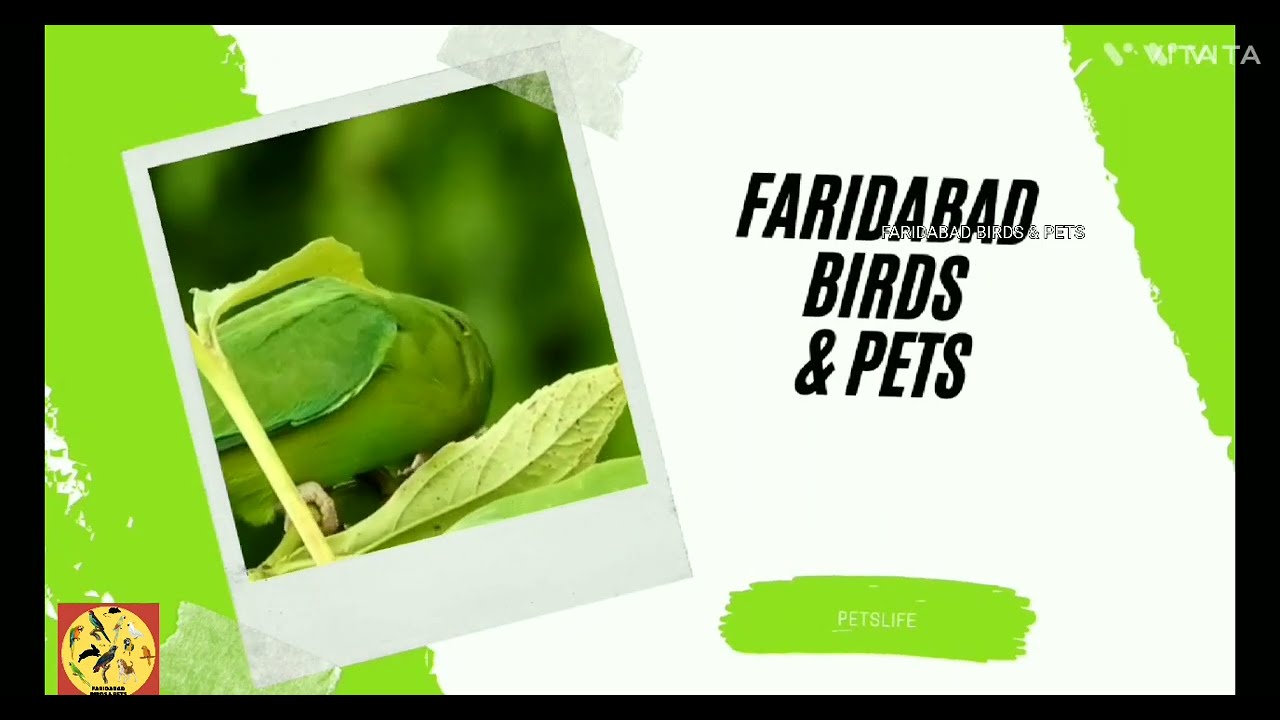The image is a black-bordered, landscape-oriented graphic with a thick white stripe running vertically through the center, flanked by green stripes in the upper right and lower left corners. Prominently displayed in bold black text on the white stripe are the words "Faridabad Birds and Pets." Beneath this, a green splotch contains the phrase "Pets Life" in white text. In the upper right corner, there is a watermark that features a 'V' and the name "Vittaya." The lower left corner hosts a distinctive red square with a yellow circle inside, depicting various animals and birds. A Polaroid photograph, seemingly taped to the background, is partially visible on the left side of the green and white striped field. This photo shows a leaf with a green, bulbous figure atop it, possibly a caterpillar or a reptile, though the image is somewhat unclear. The overall impression is that of an advertisement for pets, combining text and vivid imagery in a visually engaging yet somewhat cluttered design.